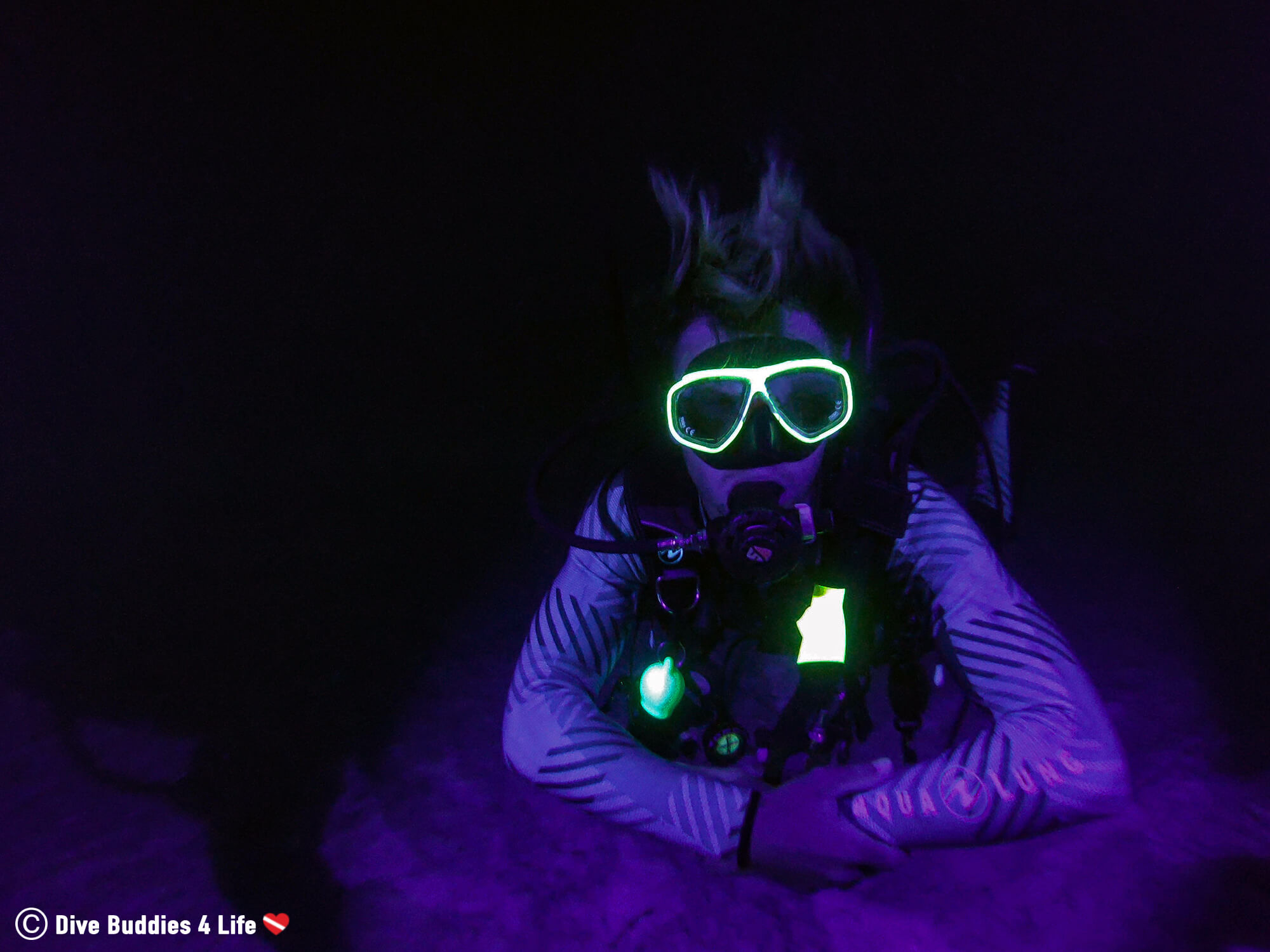In this compelling underwater scene, a scuba diver is immersed in an inky black environment with ethereal blue and purple lighting accentuating the darkness. The diver is fully equipped, wearing a striking white long-sleeve bodysuit adorned with iridescent, shimmery diagonal stripes, and the words "aqualung" emblazoned in pink on the left arm. Their gear includes a mouthpiece connected to tubes extending into the abyss, a chest pack with glow-in-the-dark features, and additional equipment strapped around their shoulders. The diver's neon green goggles, which seem almost electric, frame their face and illuminate brightly, providing a stark contrast to the murky surroundings. The movement of their hair confirms the underwater setting, while they rest against a rock. Notably, a neon light clipped to their belt by the air tanks adds a further touch of luminescence. The lower left-hand corner of the image prominently displays the text "Dive Buddies for Life," accompanied by a small copyright symbol, a red heart crossed by a white line, and the number four.